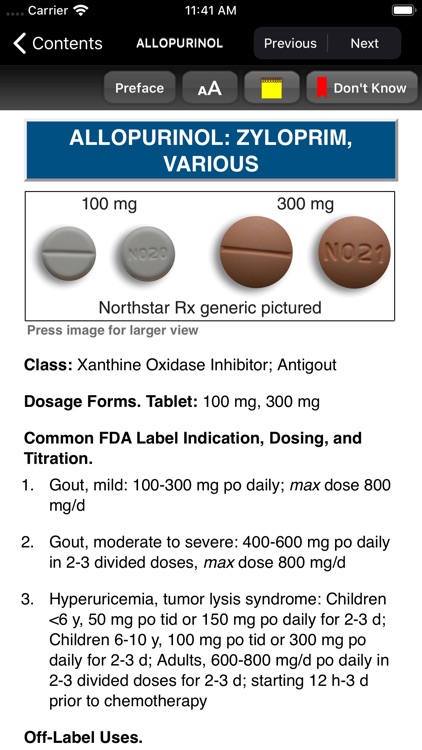The image showcases a cell phone screen displaying detailed information about the medication Allopurinol, commonly known by the brand name Xyloprim. The screen has a black border at the top, with the carrier name and a wireless signal icon on the left, the time "11:41 AM" in the middle, and a battery icon on the right. Just below this, the navigation text "Contents" is displayed alongside a left-pointing arrow, along with options for "Previous" and "Next".

The section titled "Preface" appears below, set against a blue background. Following this title, the name "Allopurinol" is presented, along with its synonyms "Xyloprim" and "Various". The screen features images of the medication, including both sides of a white pill, divided by a line and labeled with "NO20" and "100 milligrams". Adjacent to this, there is an image of a brown pill divided by a line, displaying the label "NO21" and "300 milligrams". Below these images, the text notes: "North Star RX generic pictured".

Further down, the classification "Class: Xanthine Oxidase Inhibitor, Anti-Gout" is listed, along with information about the dosage forms available: "Tablet, 100 milligrams, 300 milligrams". The screen details common FDA-approved indications, dosages, and titrations for different conditions:
1. Gout (Mild), with a specific dosage.
2. Gout (Moderate to Severe), with a higher dosage.
3. Hyperuricemia (Tumor Lysis Syndrome), with dosages differentiated for children and adults.

At the bottom, the screen lists additional "Off-Label Uses" of the medication.